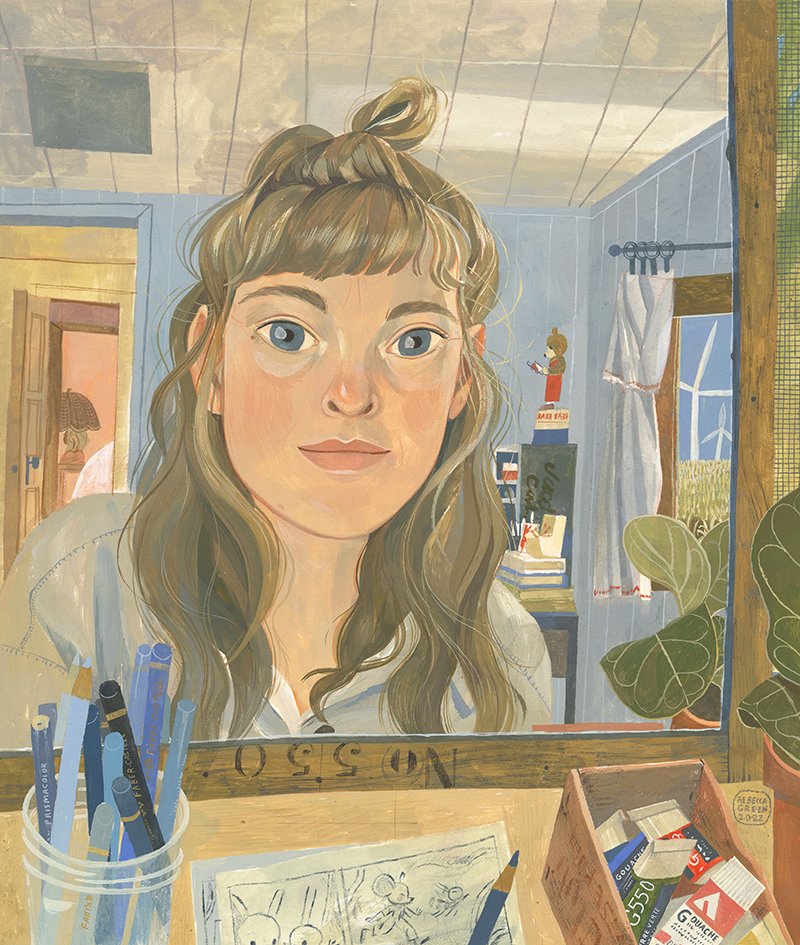A detailed painting depicts a young woman, possibly a teenager around 17 or 18 years old, sitting at a desk, gazing into a mirror with a wooden frame. The woman, with flowing wavy blonde hair, big blue eyes, and pink lips, is wearing a light blue collared shirt. Reflected in the mirror, the room is painted with blue walls and a white ceiling featuring line patterns and a vent. There is an open door, a window with white curtains, and multiple indoor plants adding to the room's decor. 

In front of the mirror, the desk is cluttered with various objects including a clear glass jar full of blue pens and pencils, a small box containing paint tubes, a vase with flowers, and a piece of paper with a sketch of a mouse, next to a blue pencil. The mirror itself has a code, "No. 550," inscribed at the bottom, adding a touch of intrigue and depth to the piece. A small stuffed bear and more stationery items are situated on a secondary desk in the background, enhancing the cozy and personal atmosphere of the scene.